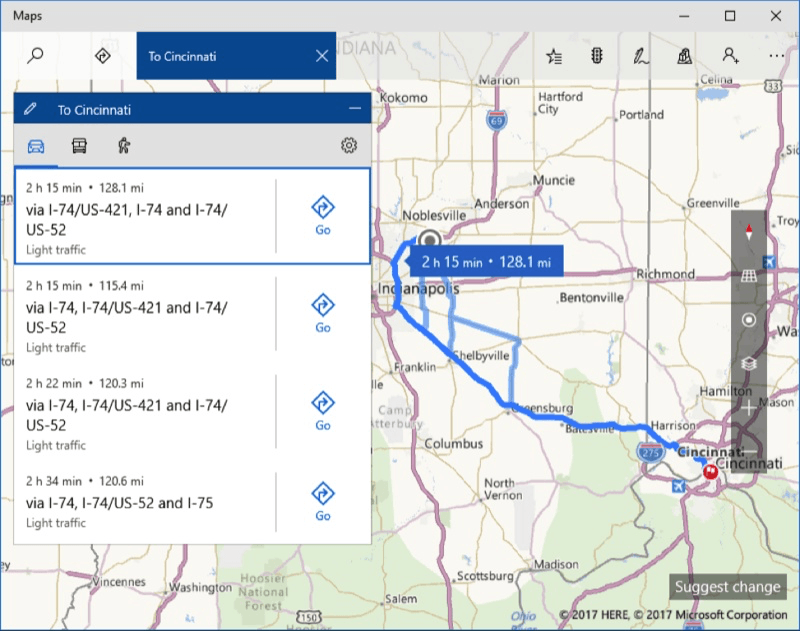The image is a digital map interface, likely from a computer or smart device, displaying navigation details. It features a thin blue border encompassing the map area. At the top is a horizontal gray bar, with the word "Maps" in black text located in the upper left-hand corner. On the upper right-hand corner of the gray bar are the minimize, maximize, and close buttons for the window.

On the left side of the interface, there is a magnifying glass icon indicating the search bar, followed by another icon, and two instances of the word "Cincinnati" in blue with a small "X" next to each, likely representing search results or waypoints.

A pop-up box appears in the interface, allowing the user to select their mode of transportation: car, bus, or walking. Currently, the car option is selected. Within this pop-up, the map provides route details, including the duration, distance, and traffic conditions. It highlights the first suggested route, indicating a travel time of 2 hours and 15 minutes over a distance of 128.1 miles, with the route itself marked in blue on the map.